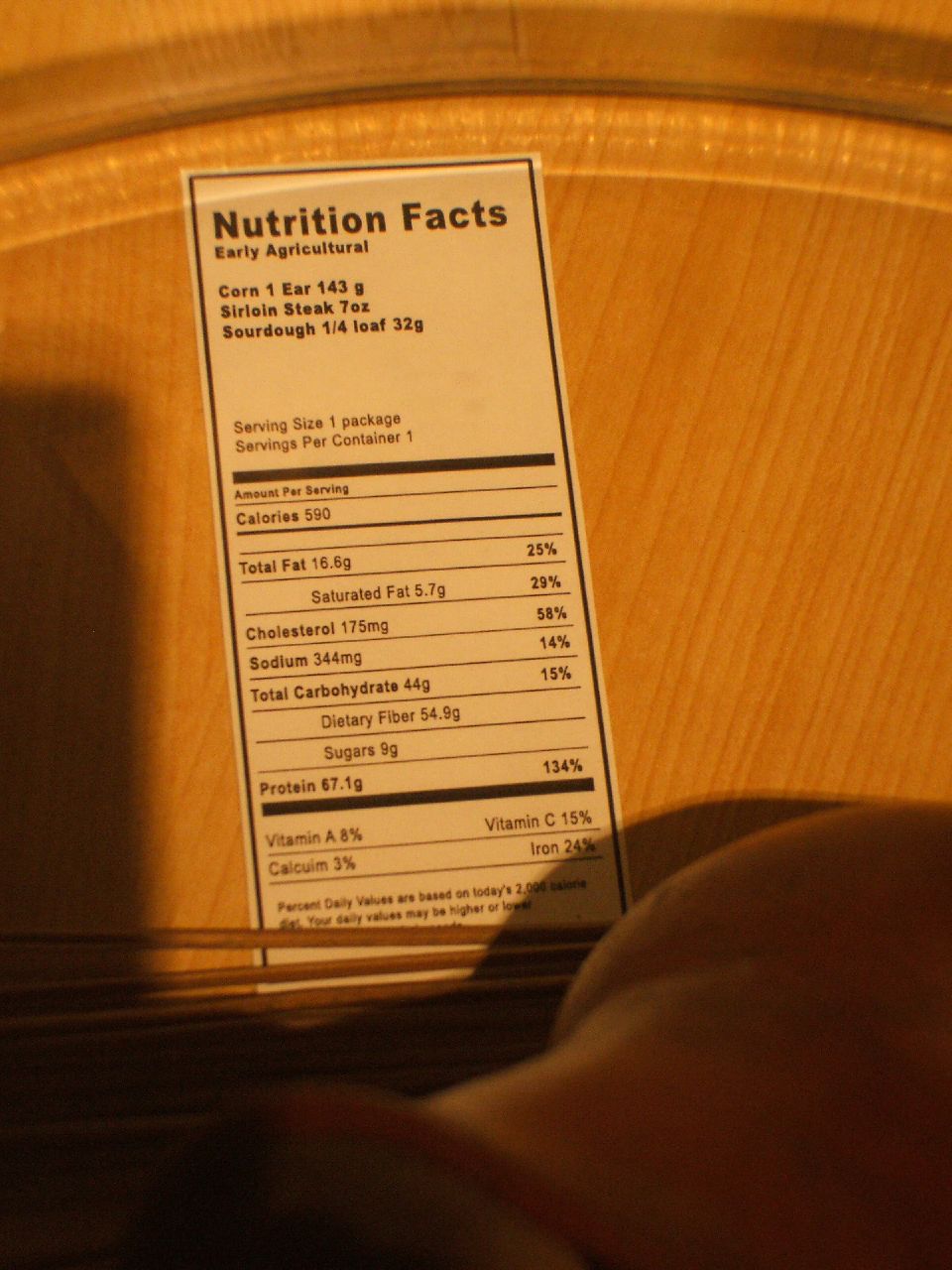This image features a long, rectangular "Nutrition Facts" sticker adhered to a round wooden board, possibly a Lazy Susan due to its raised, high lips around the edge. The sticker is white with a thin black border outlining its edges, and the nutritional information is printed in black text. At the very bottom of the sticker, three small sticks resembling chopsticks are laid horizontally. There is an apparent shadow on the left side of the photo, likely cast by the outline of a cell phone used to take the photograph.